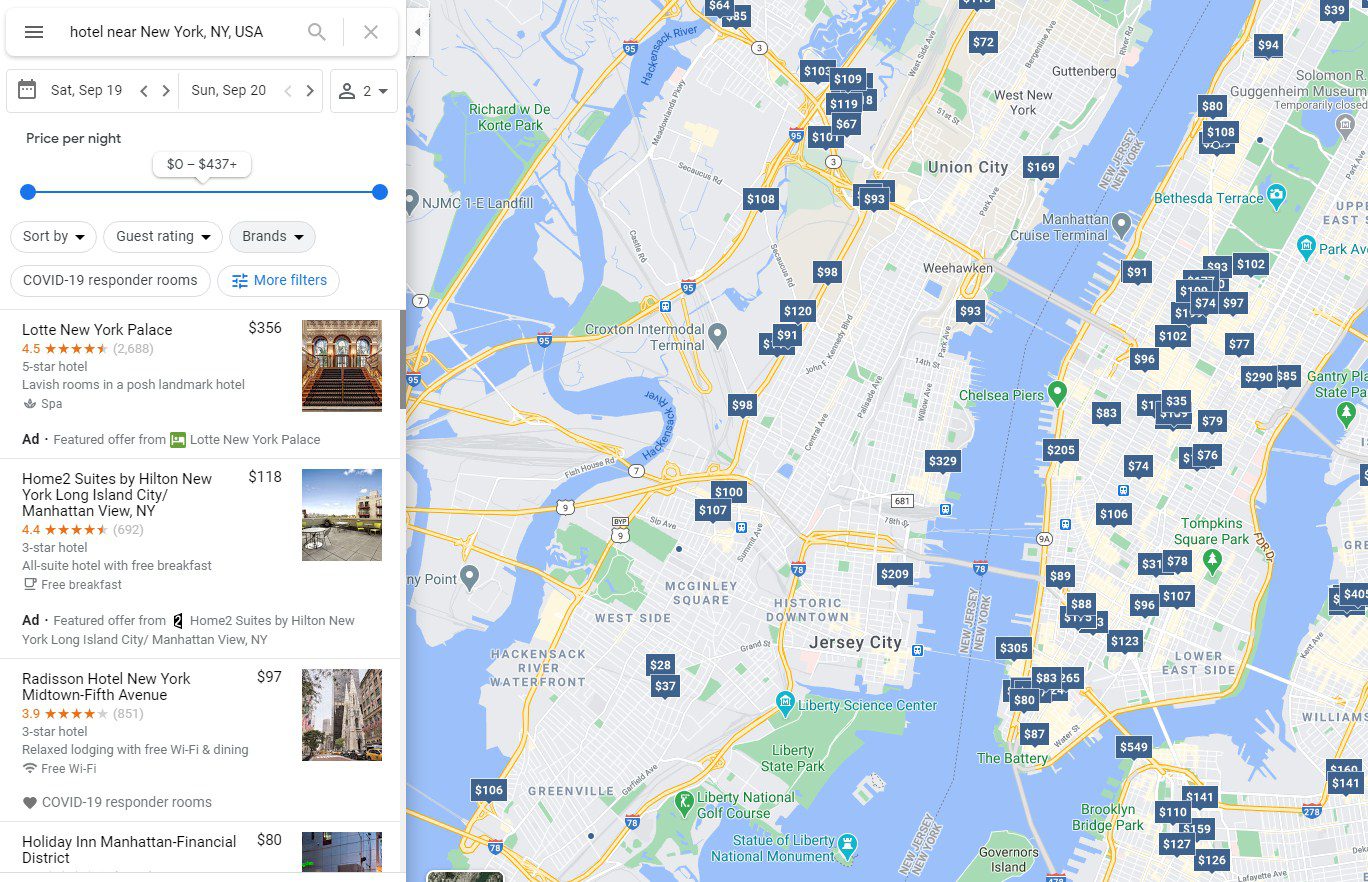The image displays a map with a search bar at the top labeled "Hotels near New York, New York, USA, Saturday, September 19th through Sunday, September 20th, for two people." It includes a price filter set to $0 to $437 per night and options to sort by "guest rating," "brands," "COVID-19 responder rooms," and "more filters."

Highlighted hotel options include:
1. **Lotte New York Palace**: 
   - Price: $356 per night
   - Rating: 4.5 stars from 2,688 reviews
   - Description: Luxurious rooms in a posh landmark hotel with a spa
   - Ad: Featured offer from Lotte New York Palace

2. **Home2 Suites by Hilton New York Long Island City Manhattan View**:
   - Price: $118 per night
   - Rating: 4.4 stars from 692 reviews
   - Description: All-suite hotel offering free breakfast
   - Ad: Featured offer from Home2 Suites by Hilton

3. **Radisson Hotel New York Midtown-Fifth Avenue**:
   - Price: $97 per night
   - Rating: 3.9 stars from 851 reviews
   - Description: Relaxing lodging with free Wi-Fi and dining
   - Note: COVID-19 responder rooms available

4. **Holiday Inn Manhattan Financial District**:
   - Price: $80 per night
   - Description: Details not specified in excerpt

The map is populated with various hotel locations and corresponding prices.